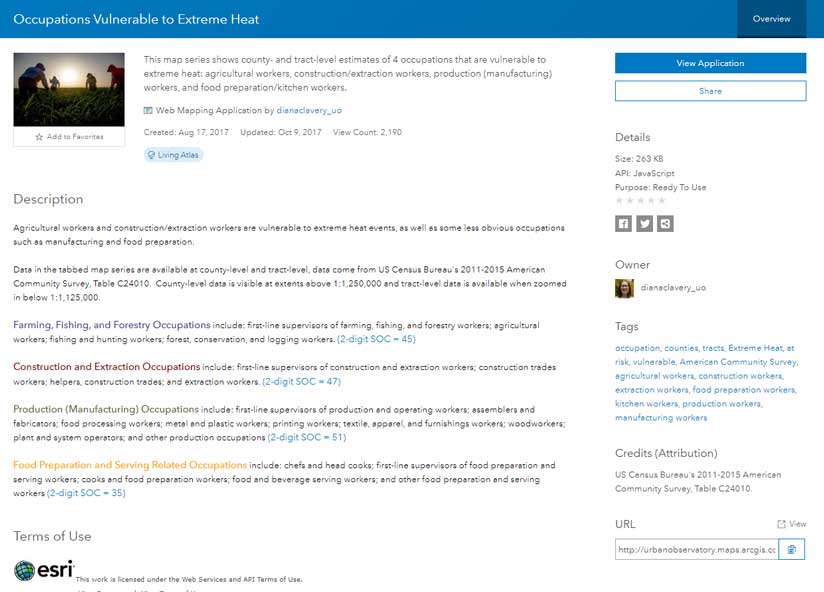Caption: 

The web page features a detailed blue border with white text at the top, stating, "Occupation Vulnerable to Extreme Heat." An overview section is highlighted in the upper right-hand corner, providing an in-depth look at various occupations affected by extreme heat. 

The page includes a small image depicting people farming under a bright sun. The main body of the text, presented in black on a white background, explains that the map series showcases county and tract-level estimates of four occupations particularly susceptible to extreme heat. These occupations are agricultural workers, construction and extraction workers, production and manufacturing workers, and food preparation and kitchen workers.

The application, created by Deanna Clavery (underscore UO) on August 17, 2017, and updated on October 9, 2017, has a view count of 2,190. The description elaborates that not only agricultural and construction workers are at risk, but also manufacturing and food preparation workers, which are less obvious but still vulnerable to extreme heat events.

Data in the tabbed web series are sourced from the U.S. Census Bureau's 2011-2015 American Community Service Table, C24010. The county-level data are visible at scales of approximately 1:1.25 million, while tract-level data can be zoomed in between scales of 1:1.125 million. 

The detailed categories of each vulnerable occupation are also expounded upon. Farming, fishing, and forestry occupations include supervisors and workers across agriculture, fishing, hunting, forest conservation, and logging. Construction and extraction occupations cover supervisors, trade workers, helpers, and specific roles in construction and extraction. Production occupations span supervisors, assemblers, fabricators, various types of workers in food processing, metal, plastic, printing, textiles, woodworks, plant, and system operators. Food preparation and serving roles include chefs, head cooks, supervisors, cooks, food prep workers, and those serving food and beverages.

Lastly, the terms of use note that the work adheres to the ESRIA web services and API terms, licensed accordingly.